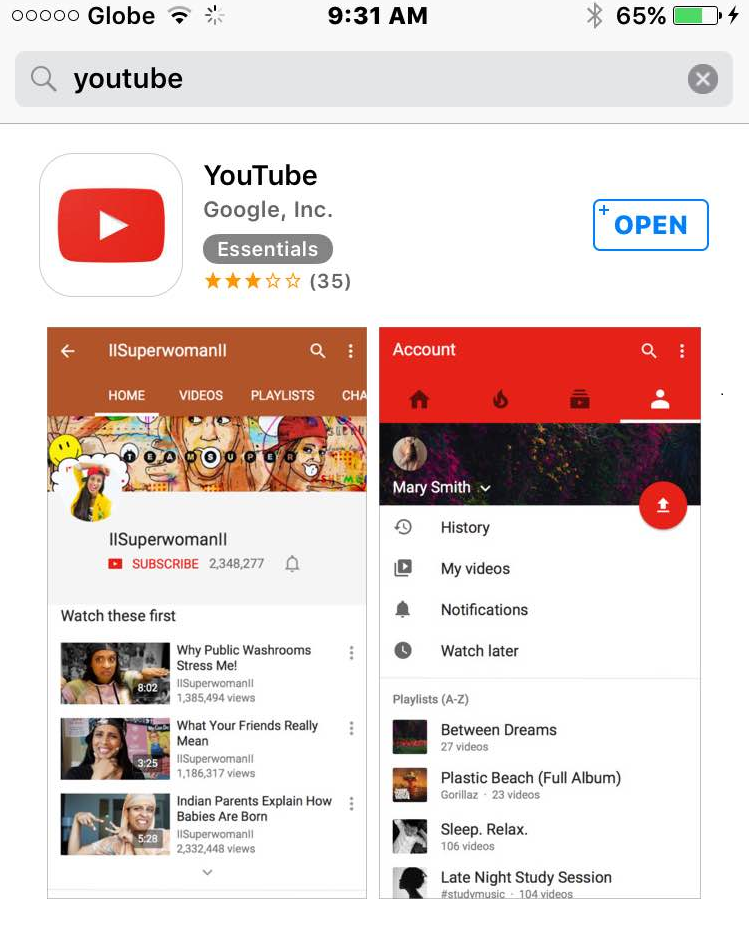This is a screenshot of a YouTube app page, displayed within a web browser. The address bar shows 'YouTube' typed into it. The status bar of the browser indicates it is 9:31 a.m., with a Bluetooth icon and a battery life of 65% visible at the top right corner. The webpage showcased is for downloading the YouTube app from platforms like the Google Play Store and Apple Store.

At the top, the YouTube brand logo and the app name "YouTube" by Google Inc. are prominently featured. An essentials tag is displayed, indicating the app's importance, along with a 3.5 out of 5-star rating. To the right, a blue "Open" button is visible for users who already have the app installed.

The page continues with two app screenshots positioned side by side. The first screenshot displays the YouTube channel landing page for 'IISuperwoman11', showing her subscriber count of 2.3 million and a bell icon for notifications. Below her subscriber count, three video thumbnails are listed.

The second screenshot showcases a Google profile for a user named Mary Smith, characterized by a red header and an avatar featuring her face. Under her name, options for 'History', 'My Videos', 'Notifications', and 'Watch Later' are listed, followed by a 'Playlist A to Z'. Near the top, there is a red circle with a white upward-pointing arrow inside it, indicative of an upload or action button.